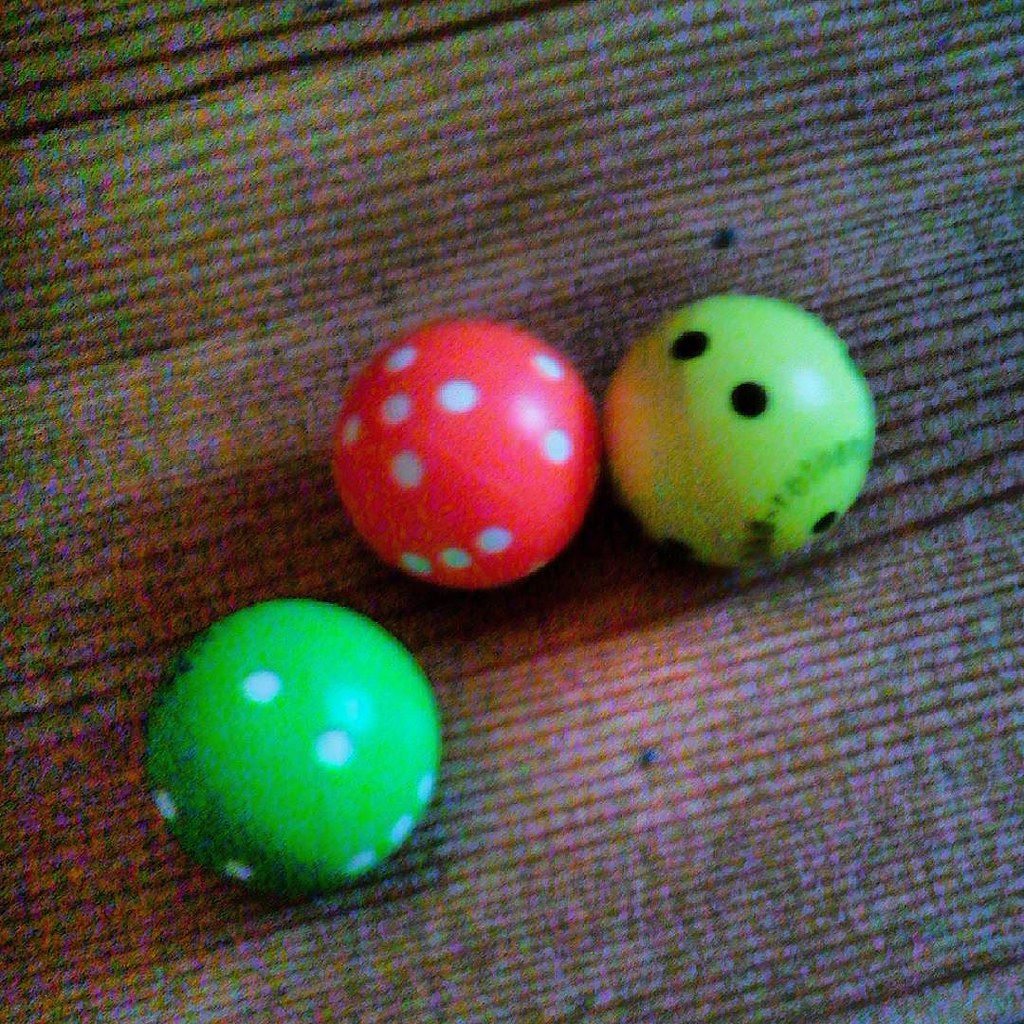This slightly out-of-focus photograph showcases three small, round spheres on a light brown carpet with distinct horizontal brown lines running across it. Each ball is perfectly spherical and similar in size, roughly comparable to marbles, creating a visually uniform set. Positioned on the lower left is a dark green ball adorned with irregular white spots, akin to the dot pattern on a six-sided die. Adjacent to it in the center is an orange-red ball also featuring white spots reminiscent of dice markings. To the right of the orange ball, touching it, is a yellow ball decorated with black dots and some illegible text. Scattered across the carpet are two small dark spots near the center of the image, adding a subtle detail to the background. Despite the blurriness, the texture of the wooden table or floor beneath the carpet is faintly visible, enhancing the image's overall detail.